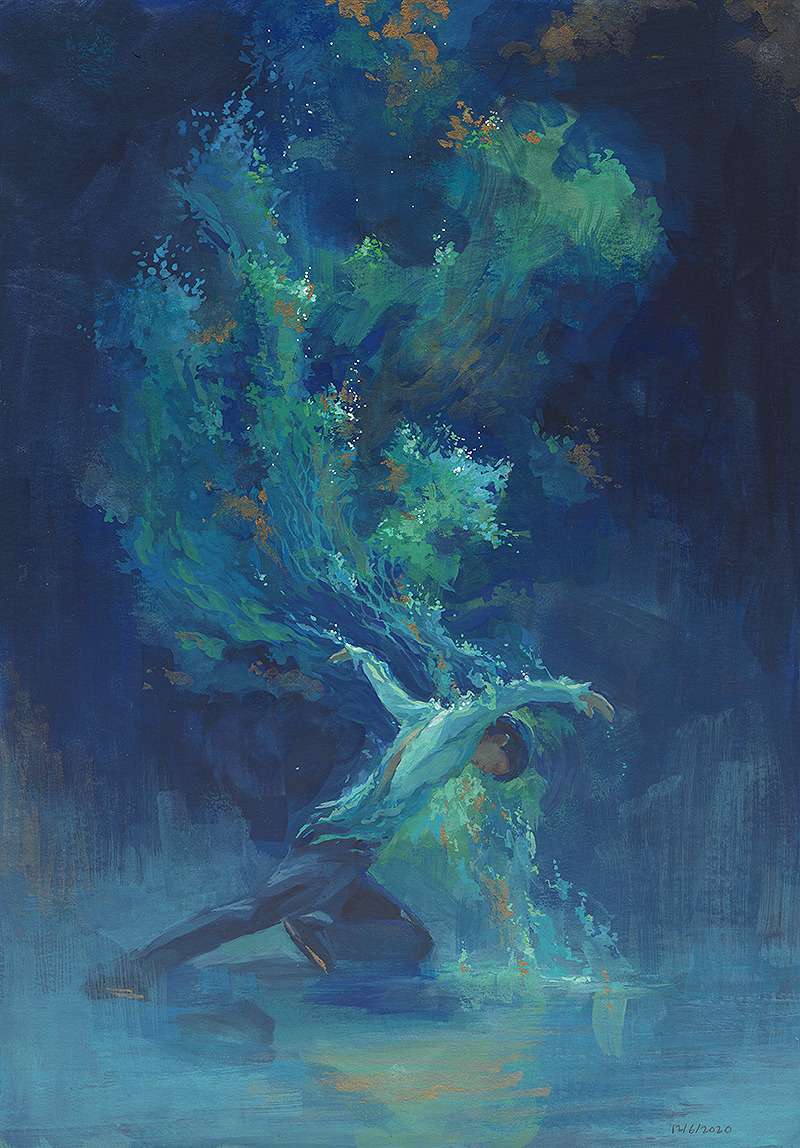The painting captures a surreal and ethereal scene featuring a man in the center, posed gracefully above a surface that could be water, ice, or earth. He is in an exaggerated, almost inhuman pose with his left knee touching down and his right leg stretched out behind him. His head is tilted backward, facing downward, while his arms curve above his head in a manner reminiscent of a bird in flight. The man's attire includes blue pants and a white shirt, and his hair has a blue tint. The background is a captivating mix of dark blues and greens, punctuated with splotches of gold and other colors. Towards the top of the painting, abstract shapes resembling tree branches with leaves emerge in hues of light green, blue, and orange. The backdrop transitions to lighter blue at the bottom, enhancing the dreamlike quality of the artwork. In the bottom right-hand corner, the date "12-6-2020" is inscribed in black text.